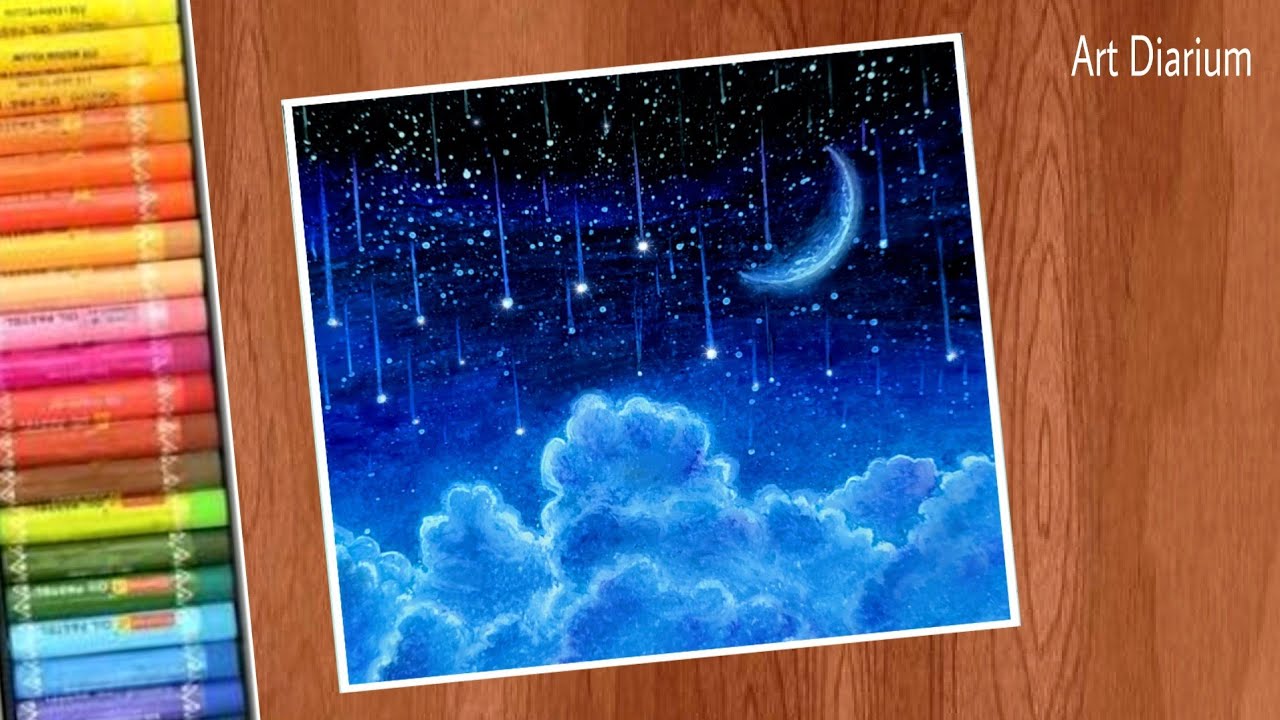The image depicts a painting of a celestial night scene, accentuated by a white border and presented on a wood grain background. The painting, which is slightly tilted to the left, is a rectangle. The top of the artwork features a black sky peppered with white spots, transitioning into a dark blue middle section displaying a bright, shadowed moon. The foreground stars appear as white dots with trailing streaks, simulating falling stars or a meteor shower. Towards the bottom, the painting lightens to blue and showcases fluffy clouds of varying blue shades with white outlines. The background is a light brown wood grain with “Art Diarium” inscribed in white font in the top right corner. On the left side of the image, there's a vertical rectangular box containing a gradient arrangement of pastels: yellow at the top, flowing through orange, red, peach, pink, brown, greens, blues, and purples at the bottom. This arrangement is angled to match the tilt of the painting, adding a colorful spectrum alongside the celestial artwork.